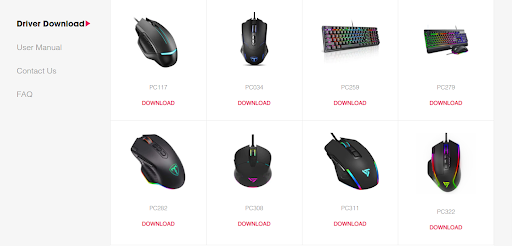Here is a cleaned-up and detailed caption:

---

This image depicts a website dedicated to PC peripherals. On the left side of the image, there is a vertical, light gray sidebar extending from the top to the bottom. The sidebar features a prominent "Driver Download" section, labeled in bold black letters with a red play button next to it. Clicking this section reveals a dropdown menu with additional options. Below the "Driver Download" section, there are links labeled "User Manual," "Contact Us," and "FAQ."

To the right of the sidebar, the main content area displays two rows of white tiles, four on the top row and four on the bottom row. Six of these tiles showcase various models of black PC mice, each equipped with RGB lighting. Another tile displays a black keyboard, also featuring RGB lighting, and the final tile presents a combo set consisting of both a black keyboard and a black mouse with RGB lighting. Each peripheral has a red download button beneath it, allowing users to download the necessary drivers for the respective devices.

---